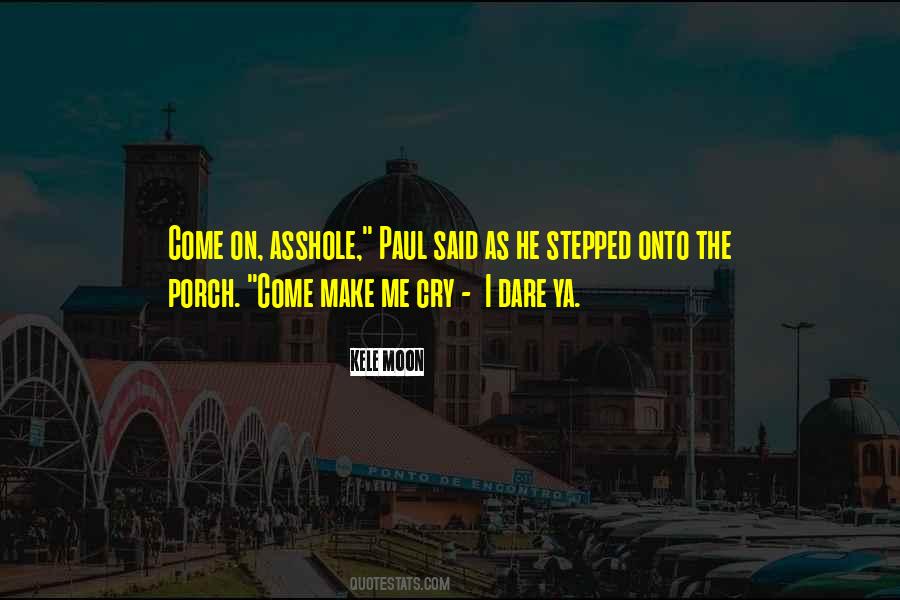The image is a darkened or faded photograph with a visually busy background that includes a large, old building, likely a church, with a prominent rounded dome and a cross on its tower. The church is surrounded by a bustling outdoor scene that appears to be either a carnival or a downtown area with visible walkways, staircases, and numerous parked cars and vans. In the foreground, there's another low building characterized by its metallic arches and a red, metal-like roof. The sky above is partly cloudy.

Superimposed prominently in the center of the image are dramatic yellow letters displaying the quote: "Come on, asshole," Paul said as he stepped onto the porch. "Come make me cry, I dare you." Below this quote, on a white background, there is black text reading, "Kelly Moon, quote stats calm." The text, placed centrally, draws immediate attention and suggests the image is intended more as an internet meme or a sharable quote than a straightforward photograph. The overall setting gives off a vacation-like vibe with people milling around, contributing to a bustling and lively atmosphere in an urban or possibly festive environment.